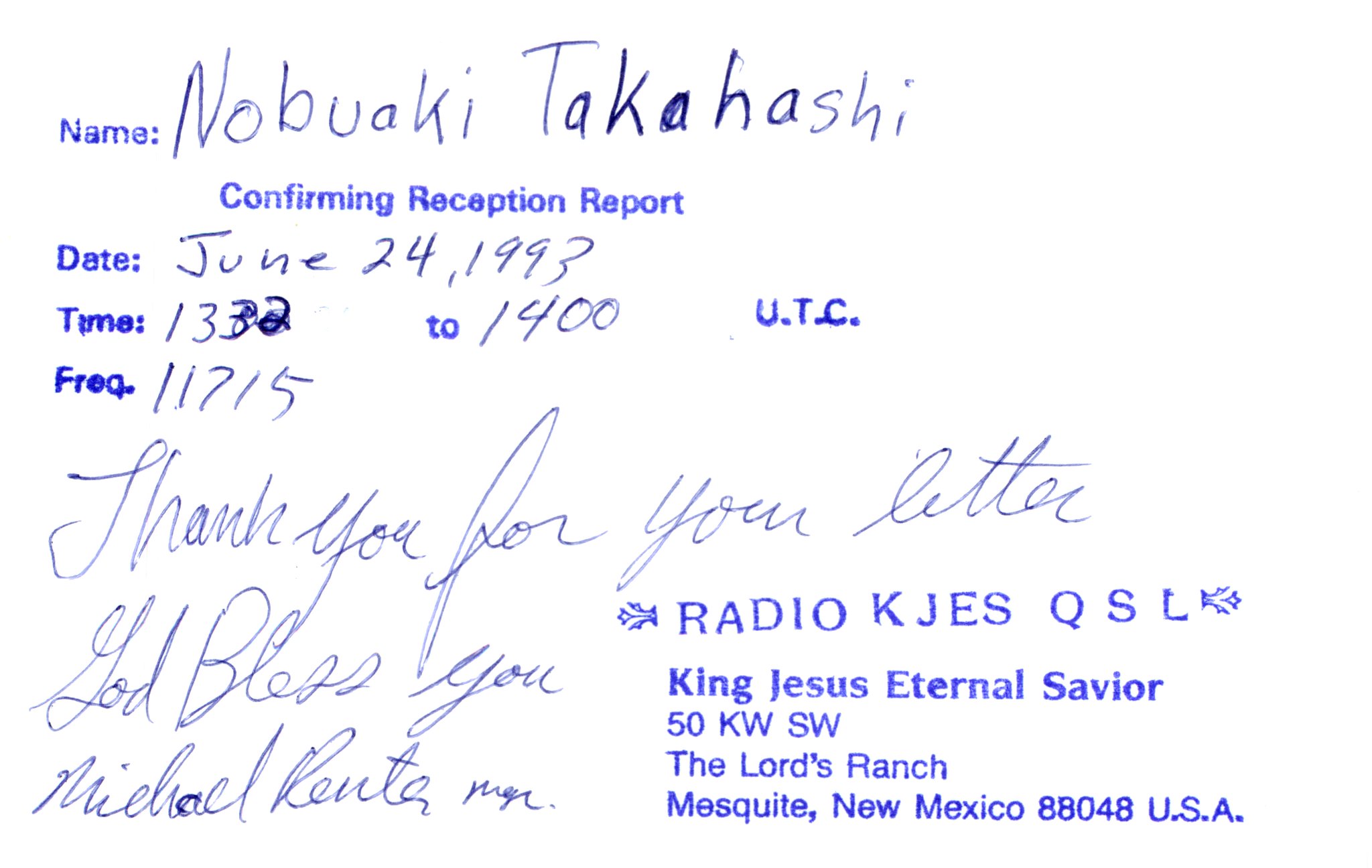The image depicts a scanned document, likely from a doctor, containing both printed and handwritten text. At the top, printed text indicates fields for a name and other information. Handwritten next to the "name" field is "Nobuaki Takashi." Below is printed text reading "confirming receipt report," followed by the date "June 24, 1993," handwritten in darker blue ink. The time fields contain printed "1332" and handwritten "1400," alongside the printed text "UTC." Below, it lists a frequency "1715," handwritten in cursive. Additional handwritten text says, "Thank you for your letter, God bless you," signed presumably by "Michael Renta, manager." The document also features a printed stamp at the bottom right with the text "Radio KJES-QSL, King Jesus Eternal Savior, 50 KWSW, The Lord's Ranch, Mesquite, New Mexico, 88048, USA." All the text, including the handwritten parts, is in shades of blue.